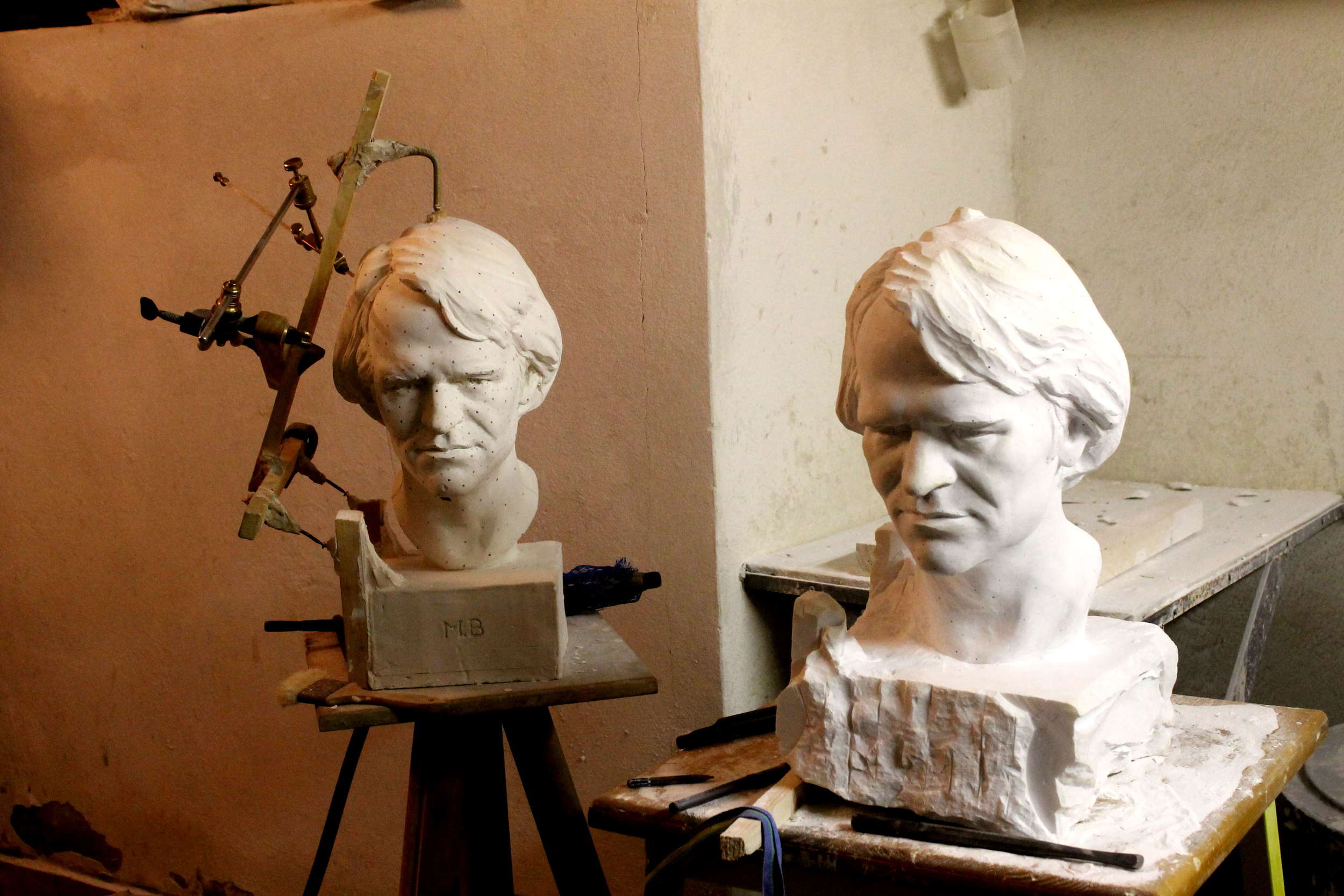The photograph depicts two exquisitely carved busts of the same male figure, likely modeled after Andy Warhol. Both sculptures capture the head from the neck up, showcasing long hair that drapes over the ears. The bust on the right is a polished, white cement sculpture placed on a small table draped with a piece of cloth, highlighting its finely detailed features. On the left, a prototype or earlier version of the same bust, possibly crafted in clay, displays the initials "MB" engraved on its wooden platform. This smaller version is surrounded by an armature, suggesting ongoing repair or measurement work. The studio setting features minimalist white walls, devoid of any individuals, creating a focused environment for the displayed art pieces.